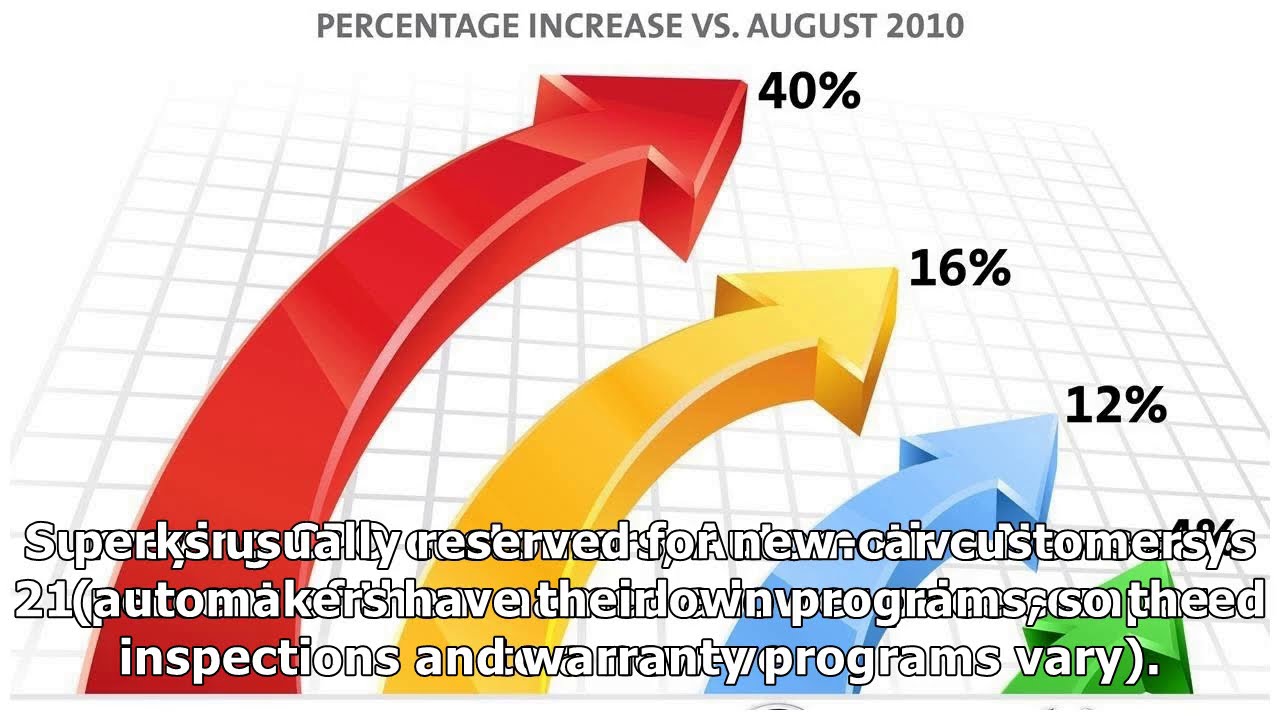The image depicts an infographic styled as a graph with multiple overlapping text layers and various colored arrows prominently placed at the center. At the top, clear text reads "Percentage Increase versus August 2010." In the forefront, a large red arrow, curving upward to the right, is labeled with "40%." Below it is a yellow arrow, also arching rightward and marked "16%." Further down, a blue arrow indicates "12%." A green arrow is visible but partially obscured by text, making its percentage unreadable. The background shows faint graph paper lines, adding to the presentation-like style of the image. The colors in the image include white, gray, red, yellow, blue, and green. Some overlapping text at the bottom mentions phrases like "reserved for new customers," "inspections," and "warranty programs vary," though it is difficult to read in full.